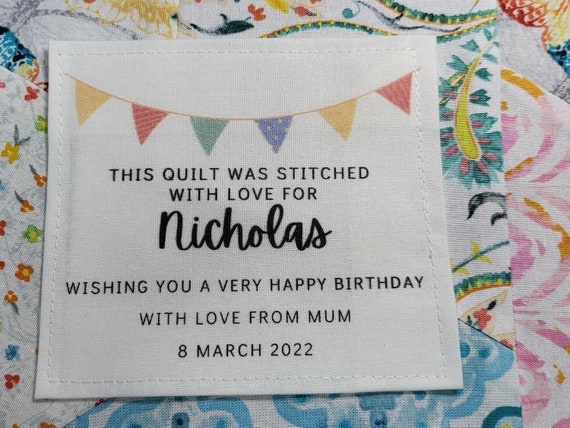This image captures a section of a vibrant, colorful quilt adorned with an array of patterns and designs. Predominantly composed of a patchwork of floral and paisley patterns in hues of blue, pink, and green, the quilt features a standout white square patch that draws the viewer's attention. At the top of this white patch is a banner of triangular pennants arranged in a cheerful sequence of yellow, red, green, blue, and repeating yellow and red. 

The patch carries an affectionate message: "This quilt was stitched with love for Nicholas," with "Nicholas" gracefully rendered in cursive, contrasting with the academic, capitalized black text of the rest of the inscription. Below this heartfelt note, the patch continues with the words: "Wishing you a very happy birthday, with love from Mom," followed by the date, "8 March 2022." The entire scene is a beautiful amalgamation of colorful designs and heartfelt sentiment, celebrating a special occasion with a personal touch.